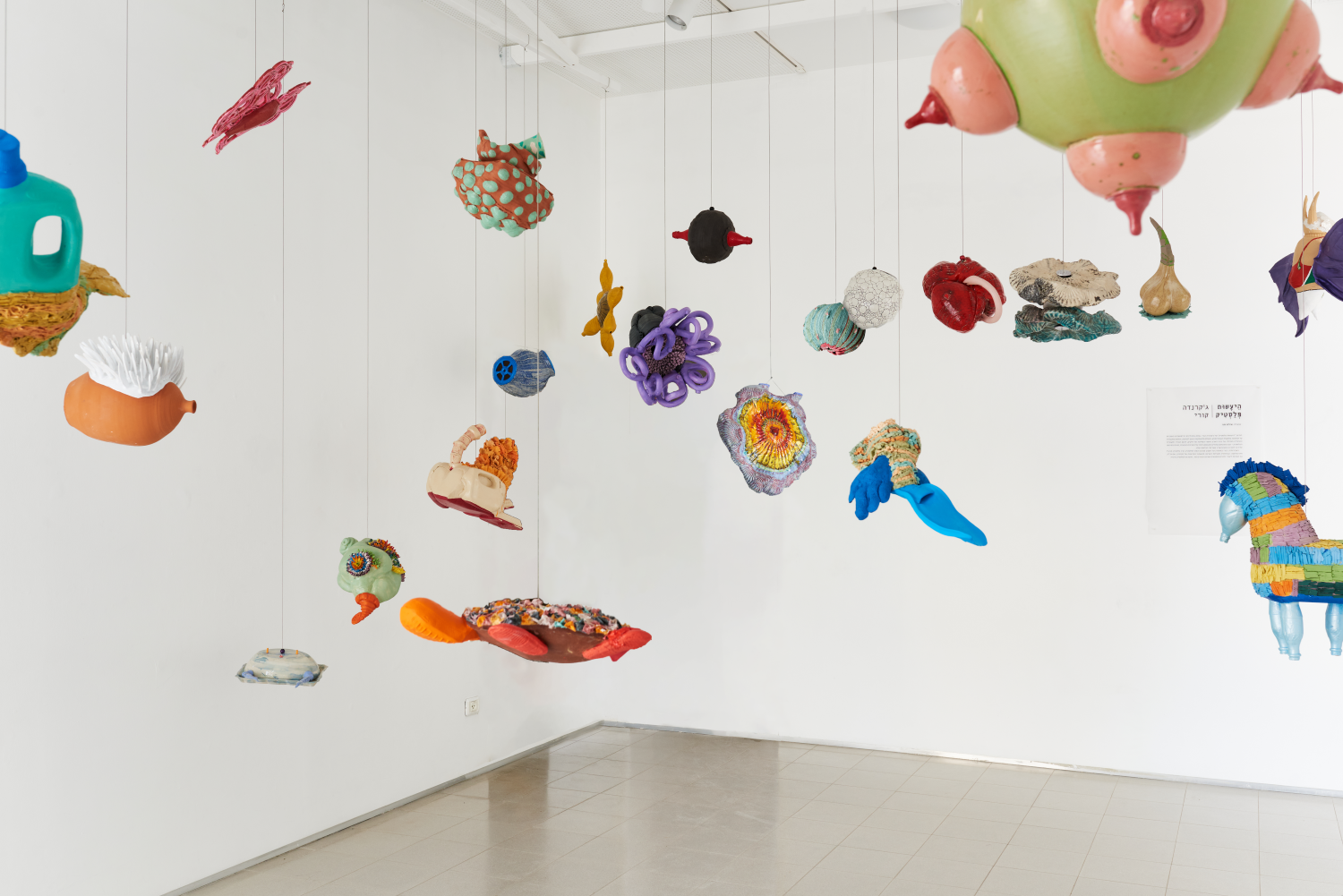The photograph depicts a bright white room with glossy gray floor tiles, empty except for a captivating art installation suspended from the ceiling by gray wires. The installation features a variety of hanging figurines and abstract sculptures in a vibrant array of colors including black, white, gray, blue, teal, green, orange, gold, yellow, pink, purple, and red. To the far right, there is a notable horse-shaped pinata, hinting at the playful and whimsical nature of the exhibit. Surrounding it are an eclectic mix of objects: some look like everyday items or animals—including what resembles a turnip, a garlic bulb, and sea creatures such as an octopus and a seahorse—while others are purely abstract shapes. A cream and aqua mushroom-like structure, a lime green sphere adorned with protruding molds resembling breasts, and a porcupine-like clay vase embellished with white spikes are among the diverse forms. One piece appears to be an aqua-colored detergent bottle with a blue lid, wrapped at its base with tan textural fabric. This striking collection of floating forms creates an engaging, almost surreal atmosphere that blurs the lines between traditional pinatas and contemporary art sculptures.